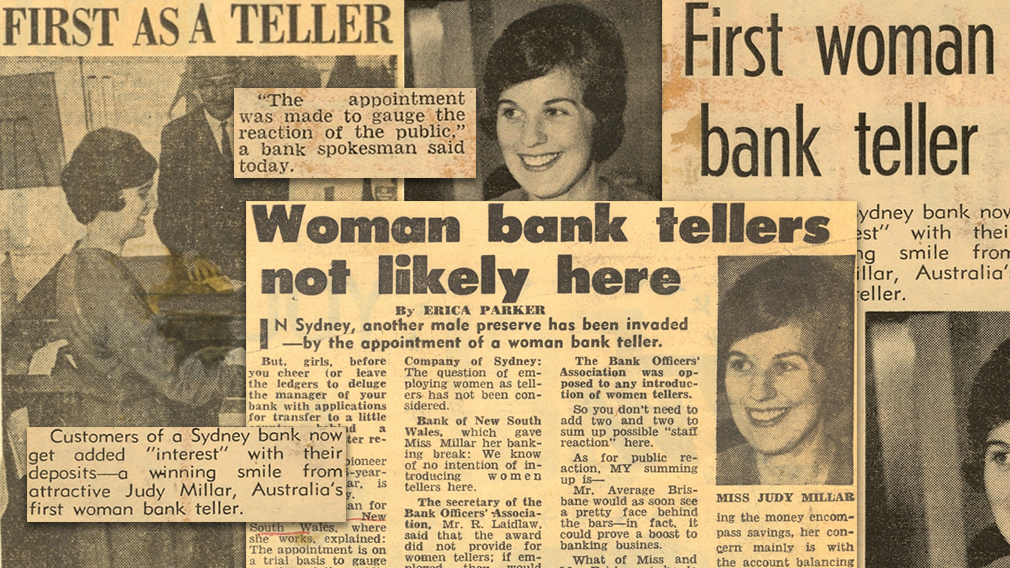The image depicts a vintage scrapbook page featuring a collage of old newspaper clippings and articles centered around the achievements of Judy Miller, the first woman bank teller in Sydney, Australia. The black-and-white images capture Judy Miller in various poses, both at the bank and smiling. Prominent headlines, such as "First as a Teller," "First Woman Bank Teller," and "Woman Bank Teller is Not Likely Here," highlight her pioneering role. The yellowed and aged pages indicate the historical significance of this collection, with detailed articles surrounding her photographs, documenting her trailblazing journey in the banking industry.